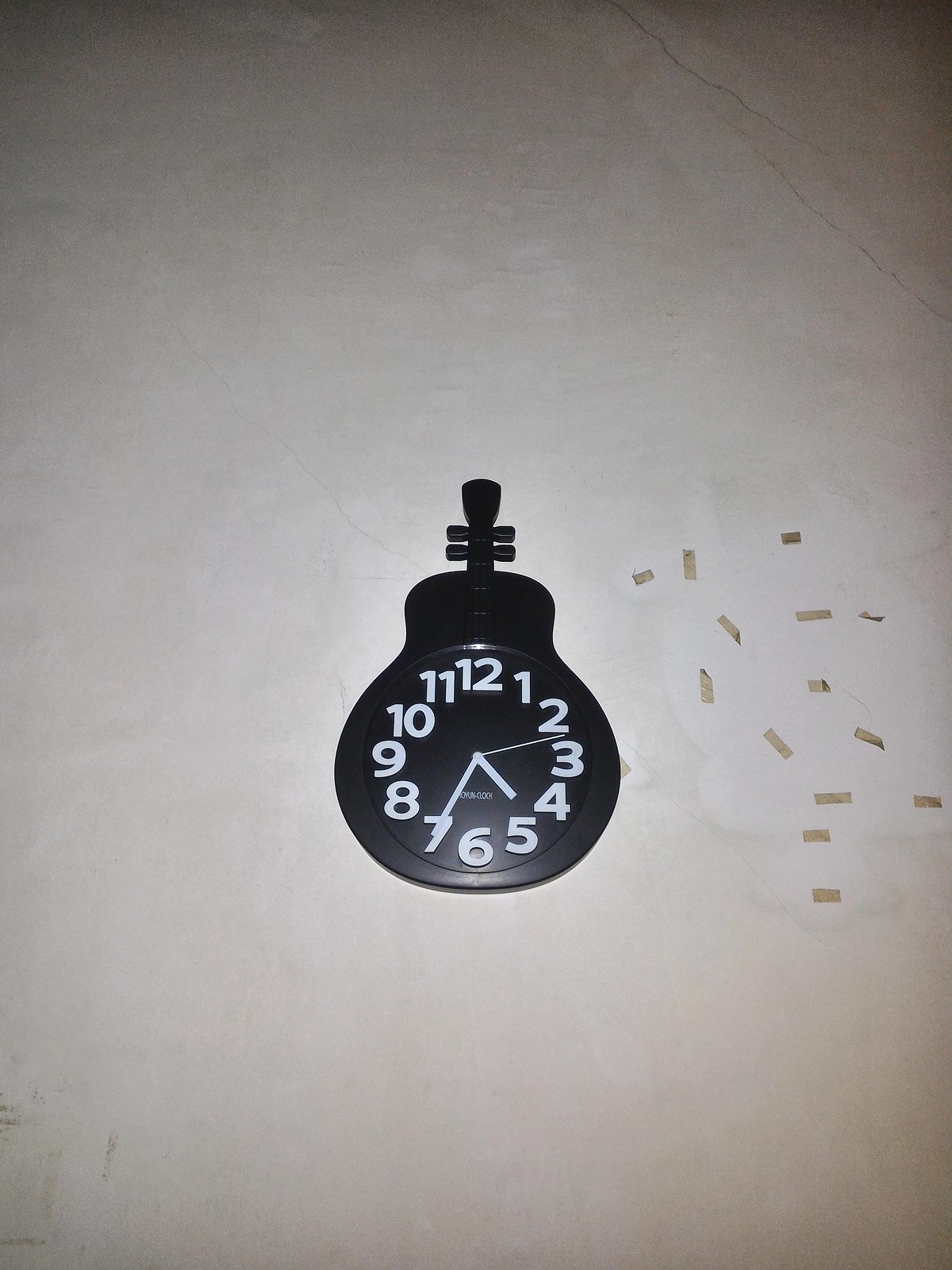In this photograph, we have a wall clock designed to resemble a string instrument, possibly a violin, guitar, or mandolin, characterized by its pear-shaped body and short neck with tuning knobs. The clock face is black with white numerals and hands, indicating the time as approximately 4:35 and 12 seconds. It features a second hand and is adorned with numbers arranged in a clockwise manner from 1 to 12. The clock is mounted on a predominantly dirty white stone ground or wall, which is somewhat weathered with visible cracks, some of which appear to have been filled but have since cracked again. There are sections of the surface that are cleaner and brighter, suggesting areas that were previously covered or less exposed to dirt. To the right of the clock, strips of tape in various directions can be seen, creating clean spots amidst the otherwise dirty surface. These strips and tape residues indicate that the wall might have been used to hang other items previously. The overall scene conveys a sense of wear and use, highlighting the distinctive and somewhat rustic backdrop for the unique clock.